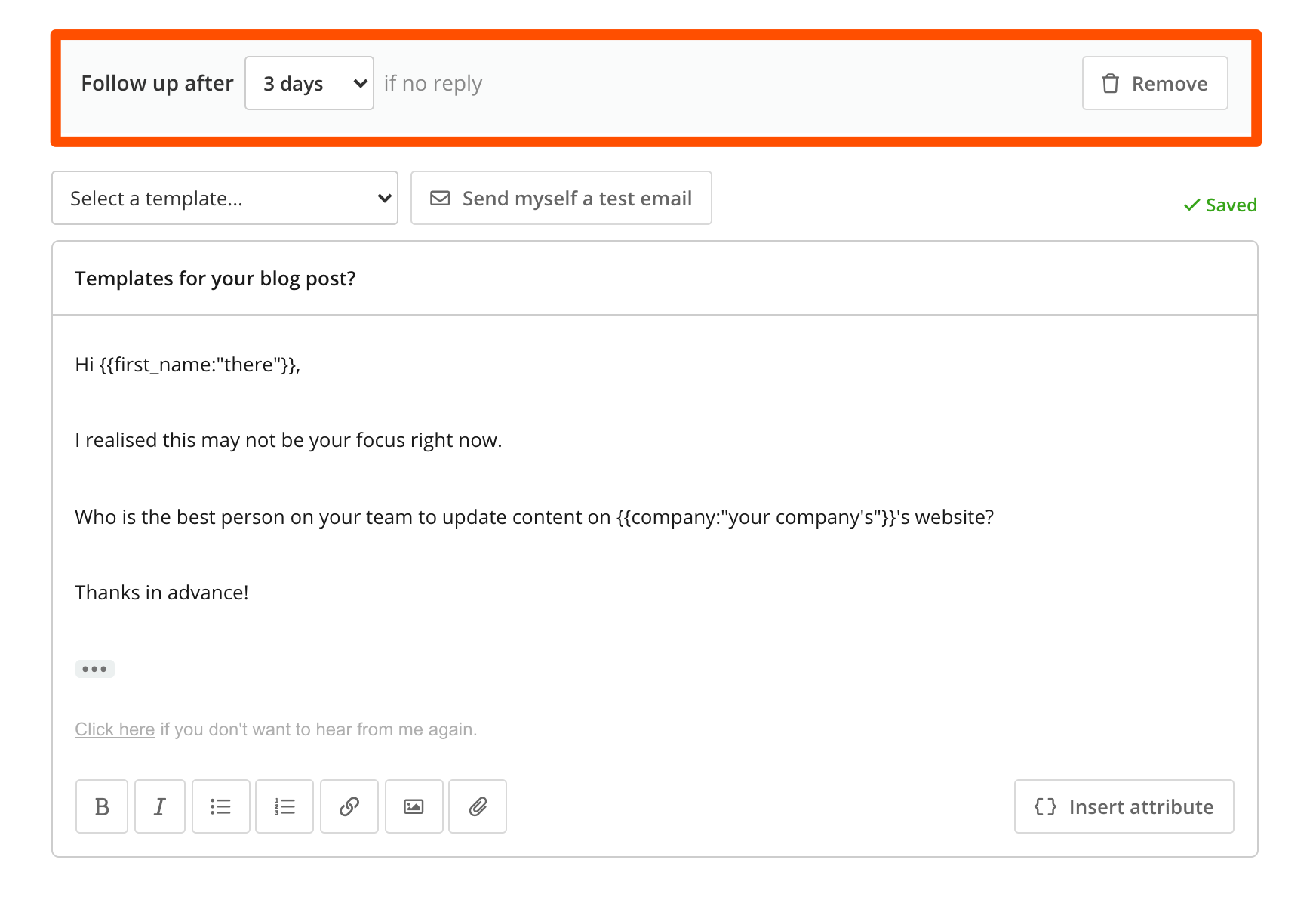The image depicts an email template customization interface designed for streamlined follow-up communications. The interface includes a customizable follow-up option set to trigger after three days of no response, with the flexibility to adjust this time frame or remove the follow-up option entirely. A section below allows users to select the type of template they wish to create and offers an option to send a test email to oneself to review the template's appearance.

In the main content window, the default template reads:

"Hi [First Name], 

I realize this may not be your primary focus at the moment, but could you please direct me to the best person in your team responsible for updating content? [Company's Name] [Website URL]

Thank you in advance."

This pre-configured template is designed to be versatile, suiting various business needs and allowing for easy reuse. Users can save multiple templates for different purposes. At the bottom of the interface, there are formatting options including bold, italics, bullet points, and numbering. Additionally, users can attach files or images to their emails, enhancing the functionality and customization of each message.